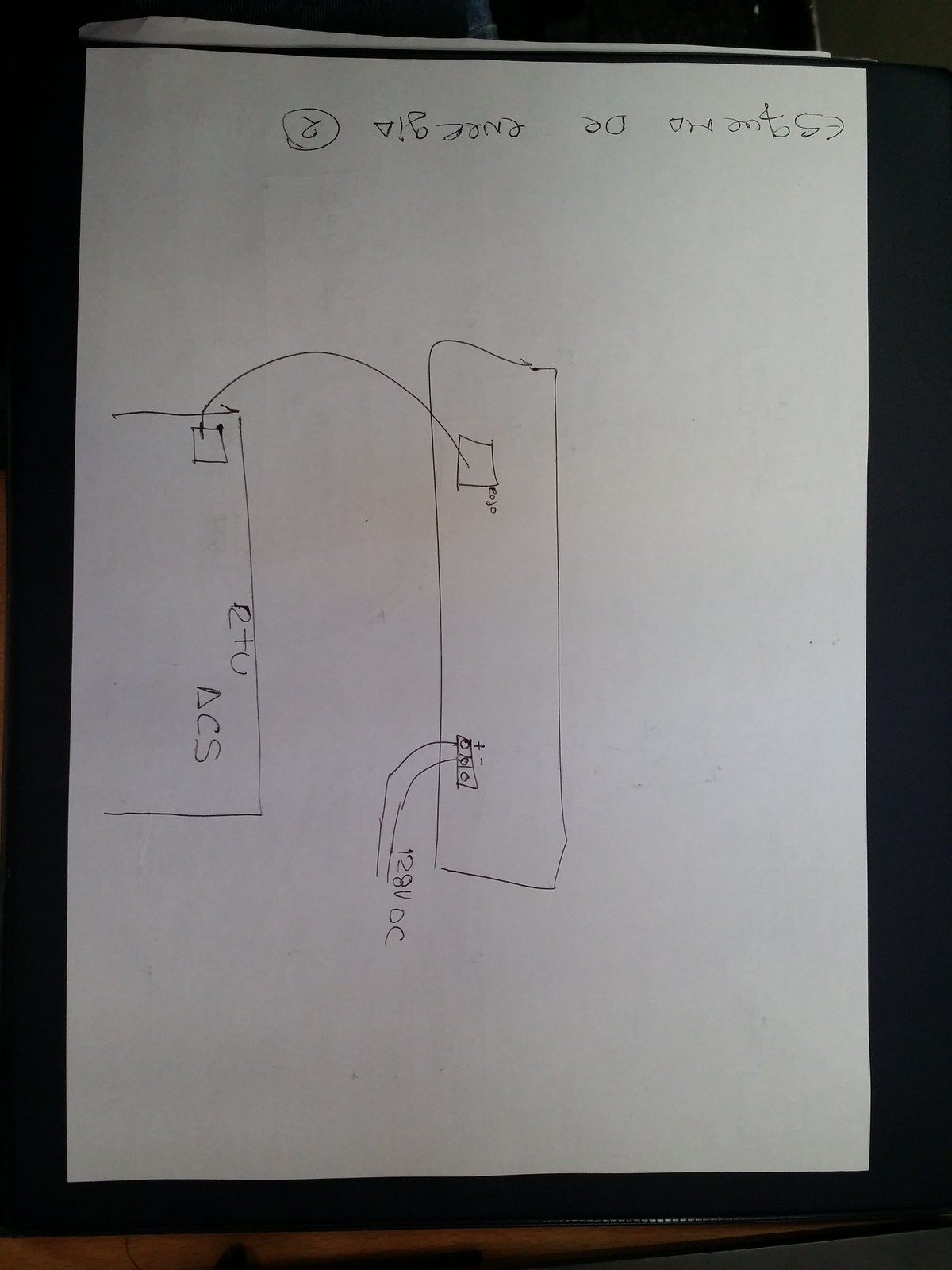The image primarily focuses on an off-white, letter-sized sheet of paper, placed in the foreground. Due to the lighting conditions, the paper appears slightly shaded with black. The top of the paper features upside-down text, which may be in Spanish. There is also an upside-down number '2' circled.

At the center of the image, there's a prominent rectangle. Within the bottom portion of this rectangle are three circles. Each of the topmost circles has lines extending from them, curving downward. Accompanying these circles, outside the rectangle, are plus and minus symbols.

One of the downward-curving lines is labeled "128VDC", possibly indicating either 128 volts direct current or 12.8 volts direct current.

Towards the top of the rectangular section, a small square with an irregular shape bears the letters "E-O-J-O" (which are not entirely clear), alongside a line leading to a three-sided rectangle with a smaller rectangle inside it. From this inner rectangle, a curved line extends to another small rectangle.

Below this, near the bottom of the page, there is additional writing that appears to be "12+U" or "T-U," though this is uncertain. On the following line, there is a delta symbol followed by the letters "C-S."